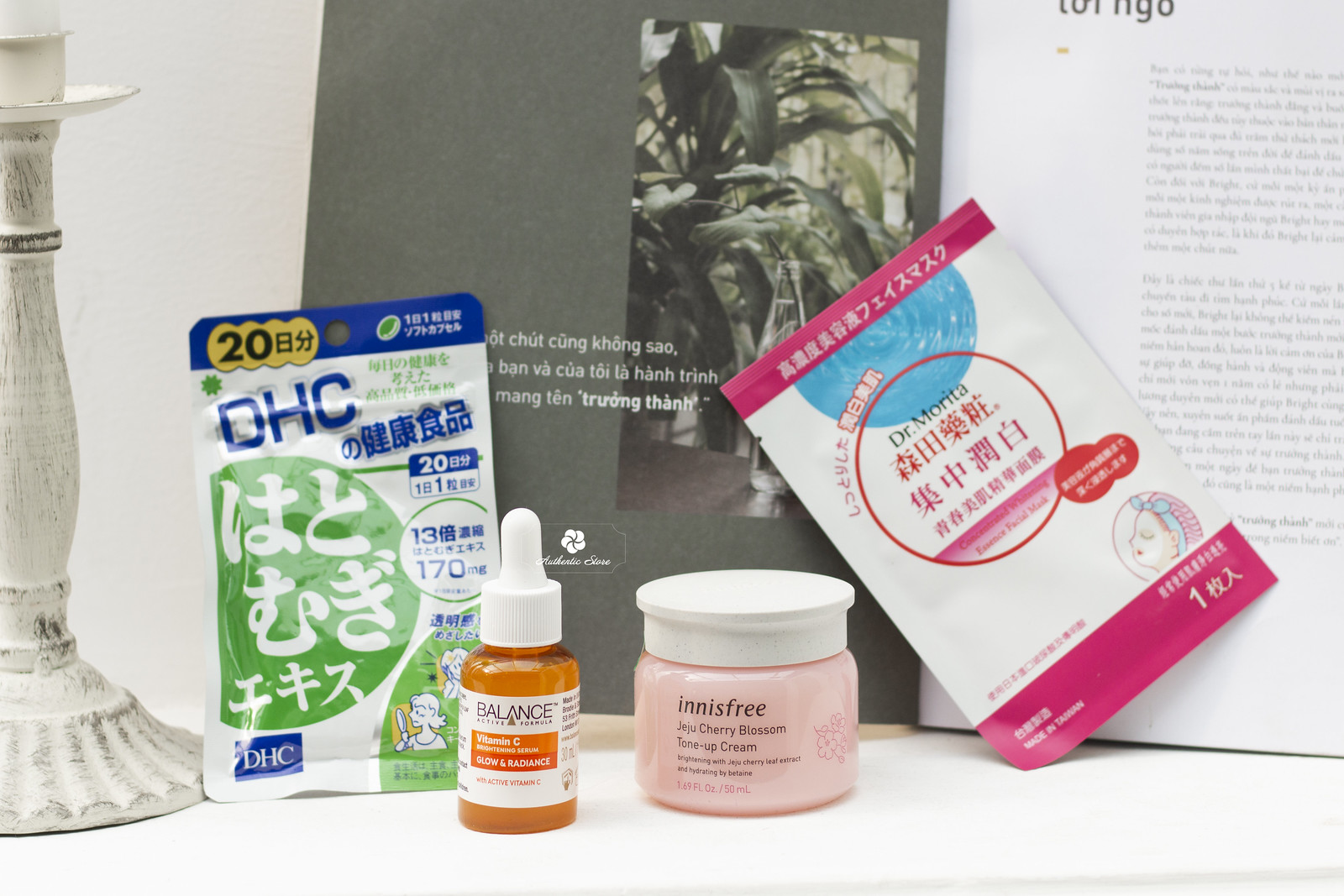The horizontal image captures a countertop adorned with various items, meticulously arranged from left to right. On the far left, partially cropped out of the frame, is an antique-style candlestick holder painted white over dark metal, giving it a vintage appearance. Immediately to its right is a package labeled "DHC" with text in an East Asian script, possibly Japanese or Korean. The package design includes green circles with white lettering and white circles with blue lettering.

Next in line is a small, brown dropper bottle with a white label and an orange rectangle indicating it contains Vitamin C. The bottle features a white stopper lid. Adjacent to it, there is a short, cylindrical jar with a white screw-on lid labeled "Innisfree Cherry Blossom Tone Up Cream," and the cream inside appears to be pink.

Positioned at a 45-degree angle counterclockwise, pointing towards 11 o'clock, is a package featuring a design with reddish borders and a white center. It displays a red circle with East Asian text, identified as "Dr. Morita," although the rest of the text is not legible. In the background, leaning against the wall, is an open book showing pages with text, possibly in Vietnamese, with the left page being predominantly gray and the right page filled with script.